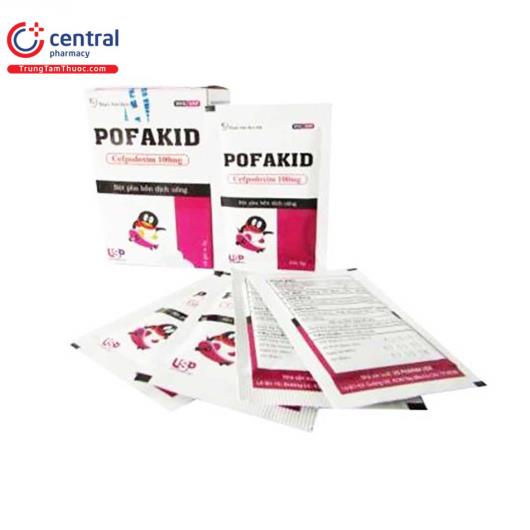The image features a white background with various packages prominently displayed in the center. In the upper left corner, "Central Pharmacy" is written in blue letters alongside a red "C" incorporating a smaller red line with a cross, serving as the logo. The main focal point is a box labeled "POFAKID" in bold black capital letters, with both a box and a plastic package shown. The package is notable for its bright pink design. On the bottom of these packages, a cartoon penguin wearing a bright pink or magenta scarf is depicted, either on a skateboard or on ice. The foreground shows four packets, two right side up and two upside down, displaying full details and information on the product. Additionally, a mention of truongthamthuoc.com in Vietnamese is seen, reinforcing the Central Pharmacy branding.